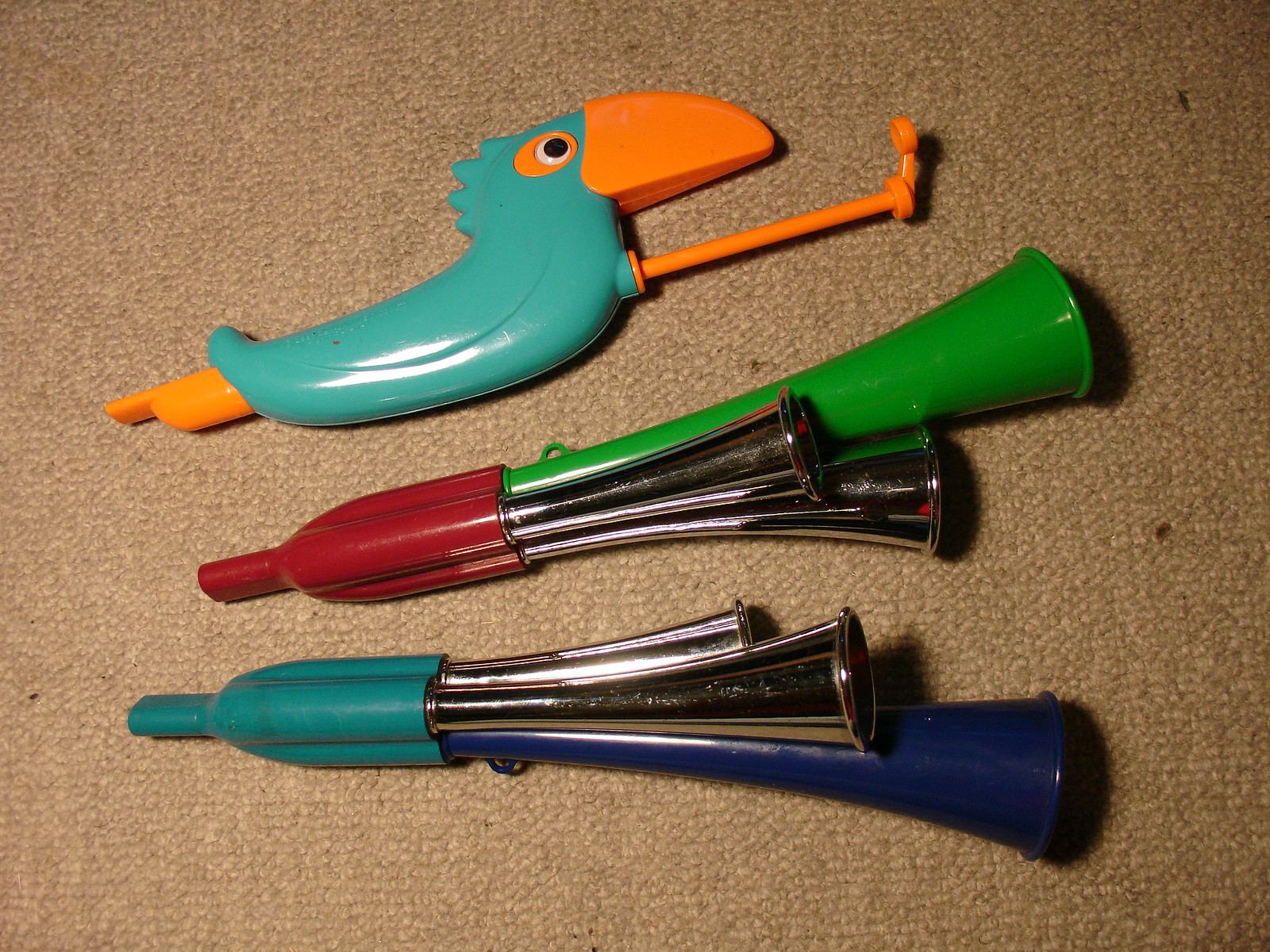The image depicts three unique and peculiar toys arranged on a beige, slightly dirty carpet with a few scattered dark spots, particularly on the right side. The toys appear to be stacked horizontally from bottom to top. At the top is a turquoise blue toucan-like bird with a prominent orange beak and an orange area around its eye. The bird also has an orange tail-like feature, and extending diagonally from below its beak is an orange rod with a small attachment, possibly a plunger for altering pitch.

The middle toy comprises a red cylindrical mouthpiece with three assembled bell-shaped tubes. The two shorter bells are metallic silver, and the longest one is a bright green. Similarly, the bottom toy features an aquamarine, turquoise mouthpiece with the same bell configuration: two shorter metallic silver bells and one longest dark blue bell. The various bells are attached to their respective mouthpieces and resemble components of a trombone.